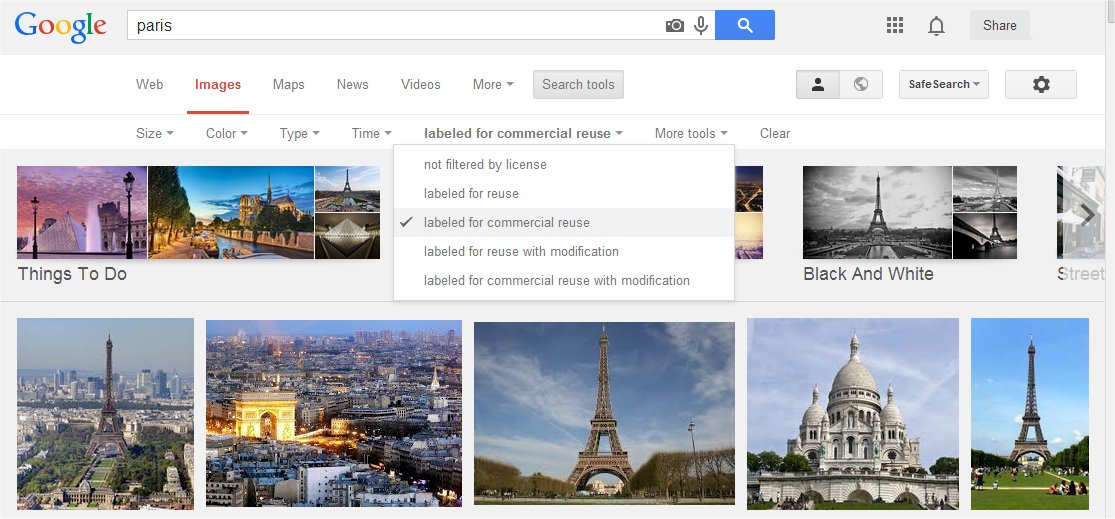The image shows the Google search results page for Paris, specifically under the "Images" tab. A dropdown menu, labeled "labeled for commercial reuse," is open, revealing various filtering options: "Not filtered by license," "Labeled for reuse," "Labeled for commercial reuse," "Labeled for reuse with modification," and "Labeled for commercial use with modification." The "labeled for commercial reuse" option is selected, highlighted in gray. Beneath the dropdown, there is a collection of images depicting Paris, partially obscured by the menu. Above the images, a smaller section titled "Things to do" is visible, showcasing more Parisian sights. On the right side of the page, there is a filter option labeled "Black and white," indicating the availability of monochrome images. The bottom of the page features a row of colorful photographs highlighting various landmarks and attractions in Paris. The classic Google branding is visible near the search bar, with its emblematic colors: red, blue, yellow, and green. Additional colors present in the images include white, gray, black, pink, orange, green, and different shades of blue and brown, capturing the diverse and vibrant essence of the city.